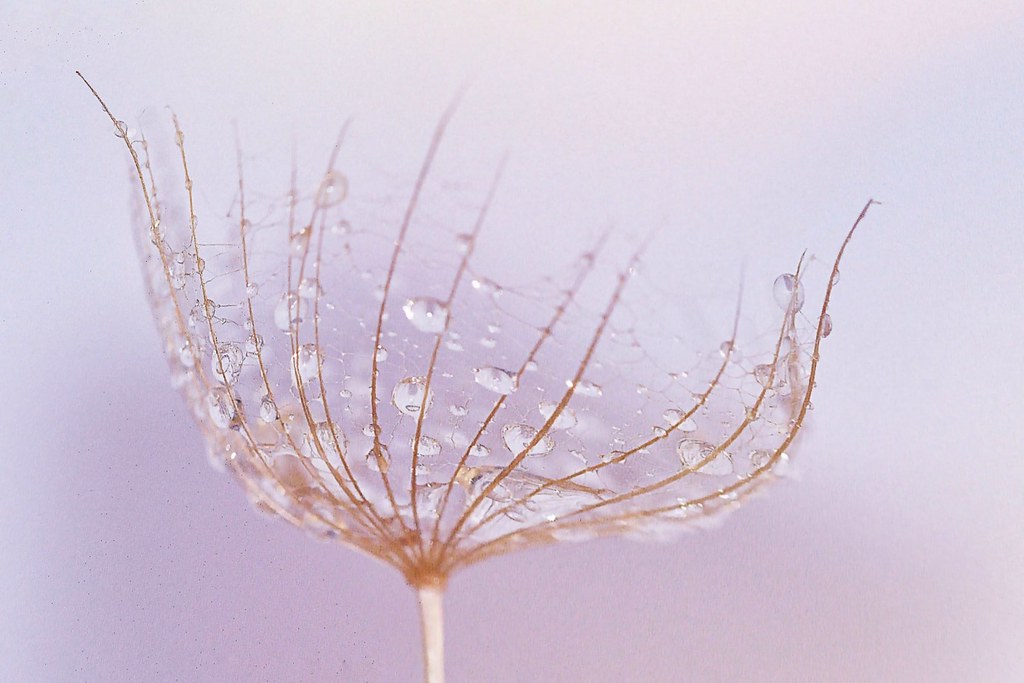This detailed, up-close image captures the ethereal beauty of a plant, resembling a dandelion that has lost its petals. The plant's narrow, beige-white stem leads upward to a collection of fine, delicate filaments that radiate outward almost like the eyelashes of an eye or the tentacles of a jellyfish. These filaments, a mix of brown and tan hues, are intricately connected by spider web-like lines, creating a skeletal structure that holds an array of glistening dew droplets. The background features a contemporary, gradient blend of light lavender, pinkish-purple, and blue hues, which darken near the plant, enhancing its fragile, rain-kissed splendor. The overall impression is that of dawn, capturing a moment of serene beauty, whether natural or artistically enhanced.